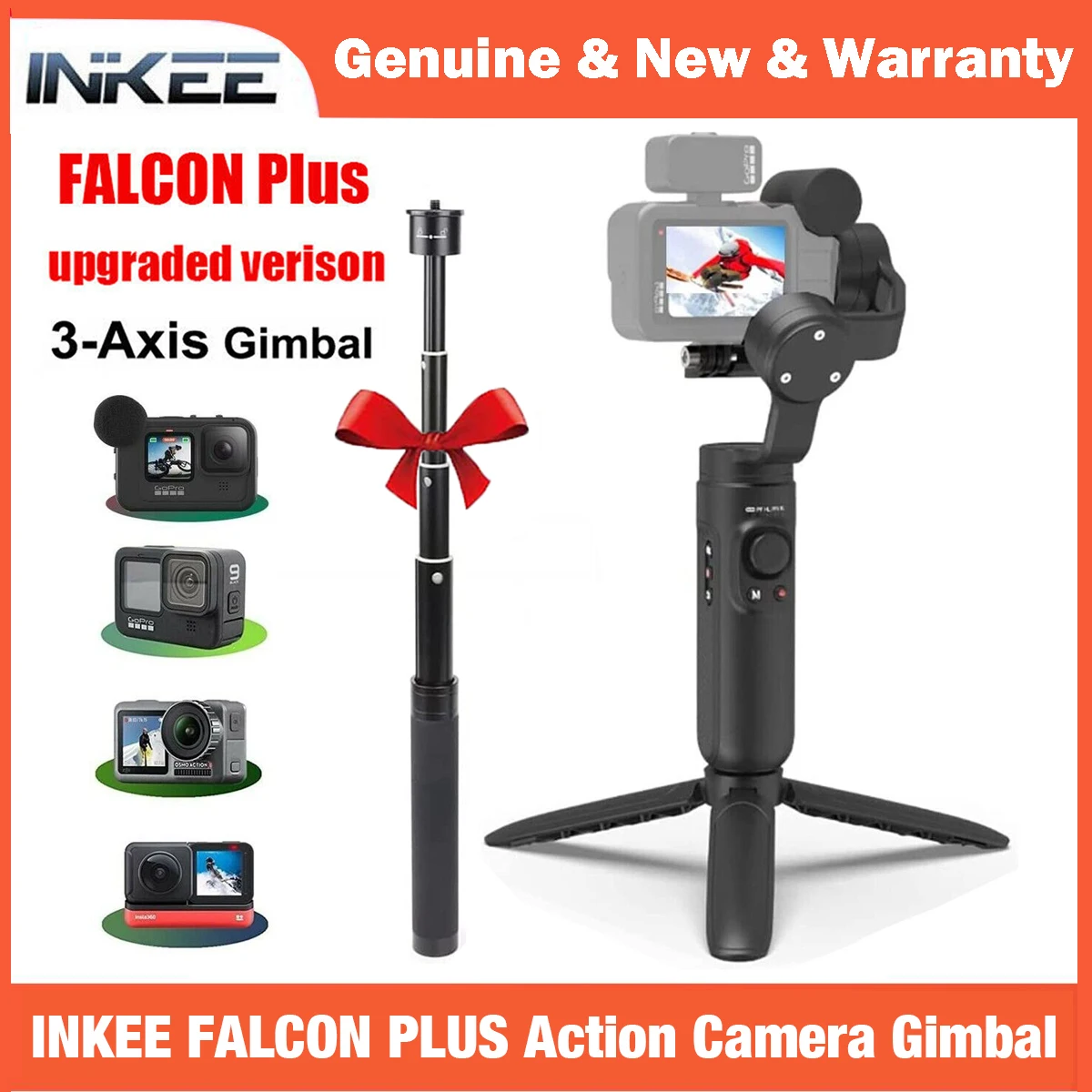This advertisement for the Inky Falcon Plus Upgraded Version 3-Axis Gimbal features a bold white background with detailed text and imagery. At the top, in white letters, the ad proclaims "Genuine New and Warranty" set against a distinctive red border. The main title, "Inky Falcon Plus," is prominently displayed, with "Upgraded Version" and "3-Axis Gimbal" beneath it.

The central illustration showcases the sleek, black metal gimbal with a red bow tied around its middle, signifying its status as a premium product. To the left, four different camera models are displayed, indicating the gimbal's compatibility with a range of action cameras. The right side of the illustration demonstrates the gimbal in action, securely holding a camera that captures dynamic footage of a man in a red jacket skiing over mountain slopes, visible on the camera's screen.

Additionally, the gimbal is shown with its three feet splayed out, highlighting its versatility as a tripod. The bottom of the advertisement reinforces the product name with the text "Inky Falcon Plus Action Camera Gimbal" in bold, white block letters. This detailed composition effectively underscores the product’s features and versatility.